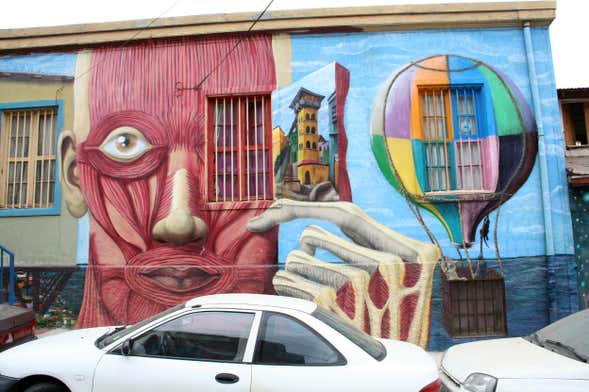In an image set in an urban landscape, there are two white cars parked tightly bumper-to-bumper on the street, with an additional dark brown car barely visible behind them. The focal point is a vibrant and detailed mural painted on the side of a one-story building. The mural depicts a person with their skin removed, showcasing their red and gray muscles and tendons. One eye is clearly visible, while the other is cleverly integrated into a window of the building, making it appear as though the window, when opened, reveals a different scene. This scene transitions into the portrayal of a tower and an architectural structure. Adjacent to this, another window is artistically transformed into a colorful hot air balloon floating in a blue sky, complete with a basket that appears to contain a small cat. The mural, with its intricate blend of anatomical detail and imaginative elements, creates a striking and thought-provoking piece of urban art.